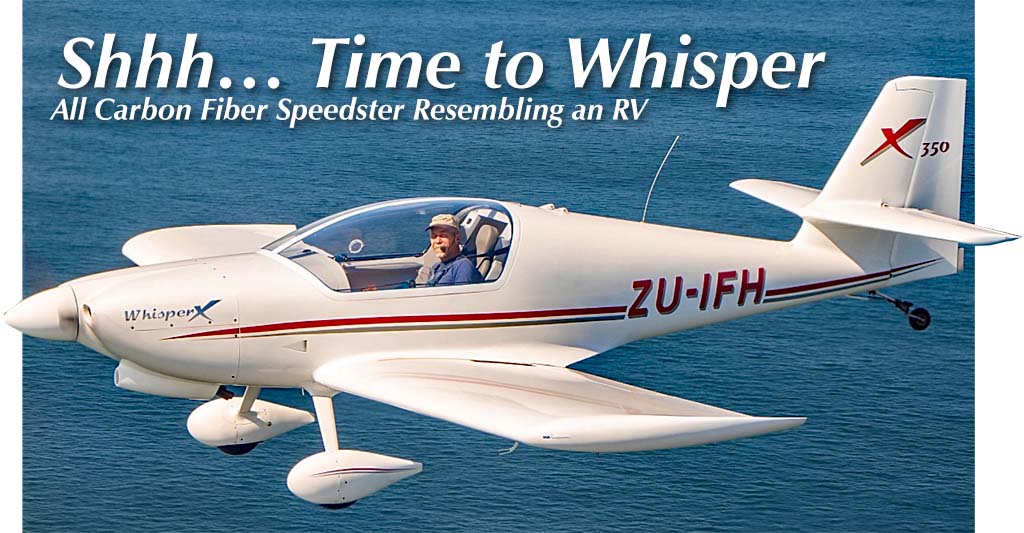This rectangular advertisement showcases a photograph of a sleek, white airplane designed for water landings, flying above an expanse of blue ocean water. The plane, identified by the letters "ZU-IFH" in bold red and trimmed in a darker color, also bears the designation "X350" on the tail fin. The fuselage features two distinct red stripes, divided by the plane's identification, running along the length of the body. The nose cone of the aircraft prominently displays the model name "Whisper X."

The advertisement is headlined with large, white text that reads, "SHHH... time to whisper," followed by the subtext, "all carbon fiber speedster resembling an RV." The aircraft itself has a clear acrylic cockpit that offers a view of the pilot, who is wearing a blue shirt, a ball cap, a headset with a microphone, and a shoulder seatbelt. This model appears to be a two-seater, evidenced by a glimpse of the another seat next to the pilot. Additionally, the plane has a unique elevator halfway up the tail, short wings, and a combination of front landing gear and a tailwheel, hinting at its water-landing capabilities.

Overall, this image presents the Whisper X350 as a modern, sport-oriented, home-built aircraft, emphasizing its lightweight, carbon fiber construction and versatile design for both air and water.